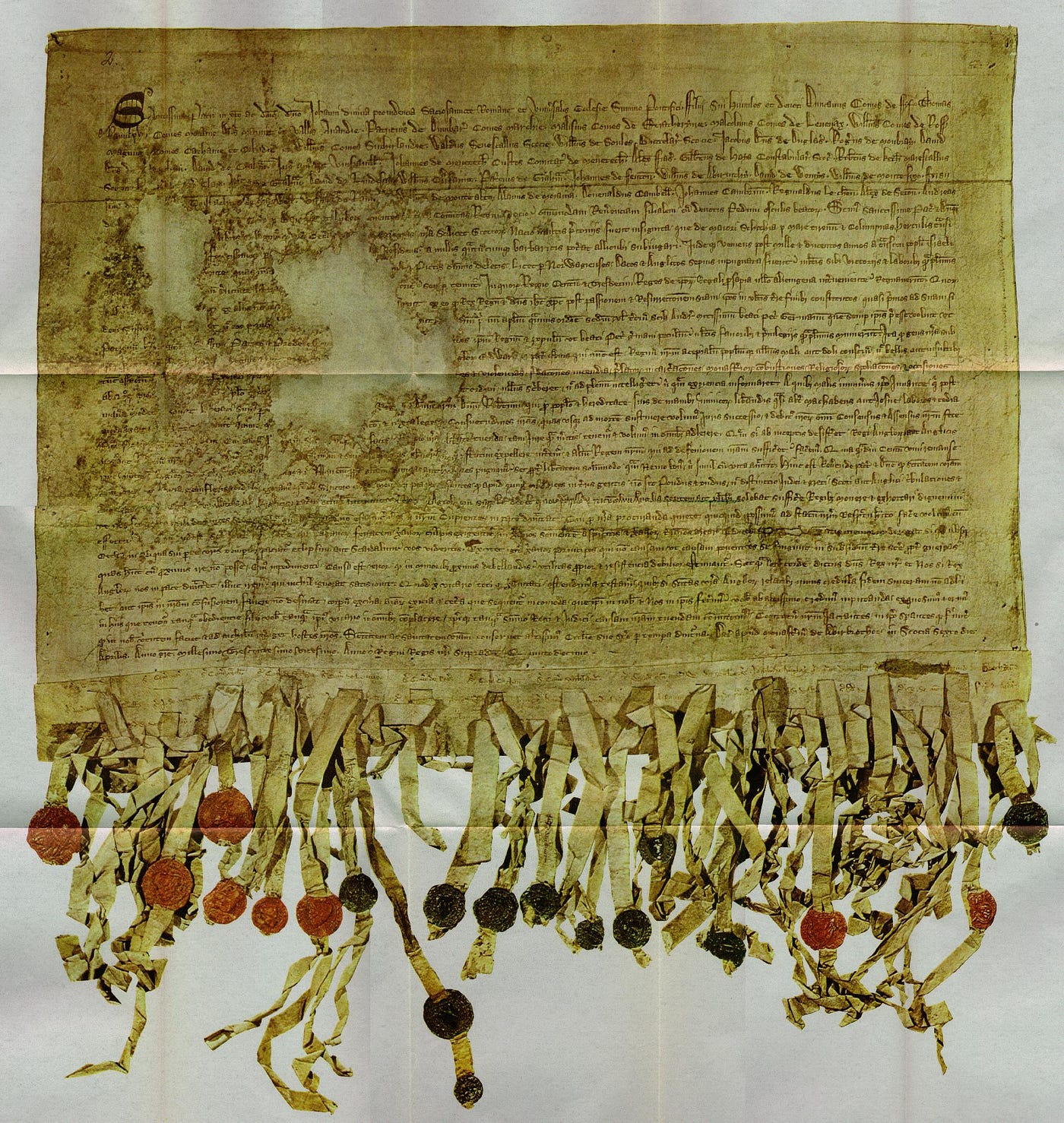This image captures a weathered and ancient piece of parchment, laid flat on a white surface. The paper is heavily aged, exhibiting a yellowing hue throughout, and is marked with notable water stains, particularly in the top left corner where some of the text has eroded away with time. The document is adorned with dense cursive writing, though the text is too small to decipher. It appears to have been folded previously, evident from the visible crease lines across its surface. At the bottom of this parchment, dozens of frayed strands of paper elegantly dangle downwards. These strands are integrated with the parchment, seemingly cut and pulled through to form a cohesive design. Each strand is tipped with either a red or black circular ornament, adding a distinct detail to the overall aesthetic. This intricate piece of artwork merges the aged elegance of the parchment with a unique, tactile embellishment.